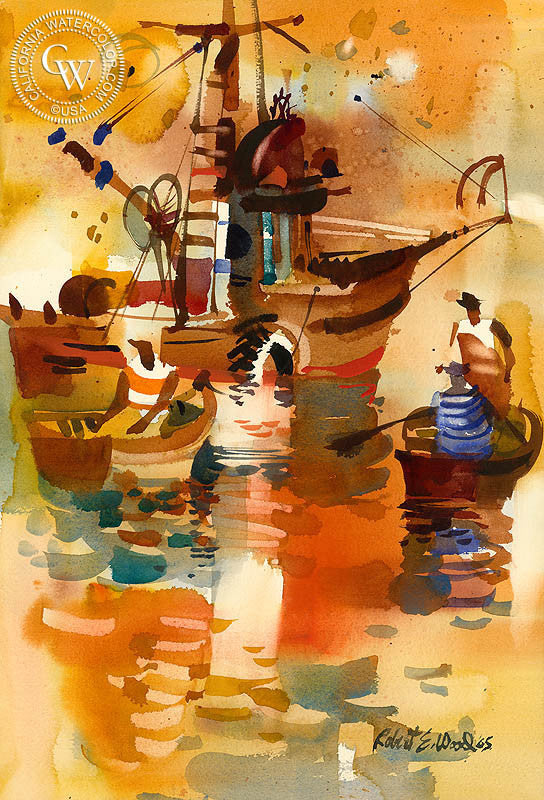This vertically rectangular watercolor painting integrates vivid digital elements, featuring a vibrant color palette with predominant shades of orange, yellow, and cream, blurring the distinction between sky and water. The composition includes a large, somewhat indistinct sailing ship, painted in brown, green, and yellow hues, positioned in the background without visible sails. In the foreground, two smaller rowboats are depicted. The boat on the left, painted in light brown with yellow and white accents, contains a solitary figure with brown skin, dressed in white and orange. On the right, another rowboat appears in brown and dark green, carrying two figures; one in blue attire and another in brown and white clothing. The figures are minimally detailed, rendered as simple streaks and blots. At the top left corner, a white circular emblem with "CW" at the center is overlayed, encircled by the text "California Watercolor Com USA." The bottom right corner bears the artist's signature, "Robert E. Dodes," in dark blue handwriting.